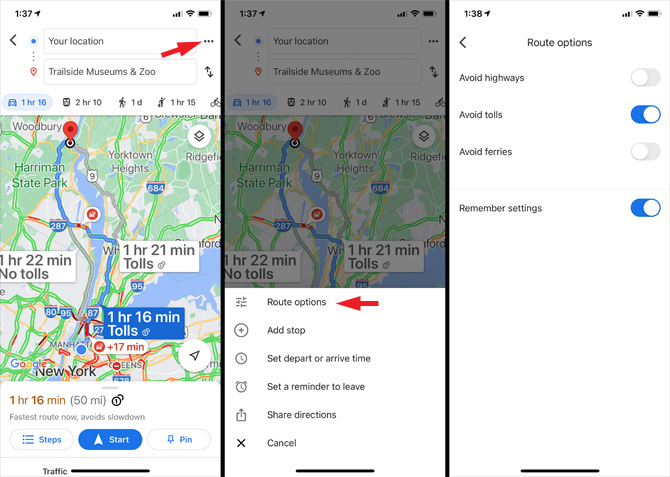The image consists of two Google Maps screenshots placed side by side. Both screenshots show a route between two locations. 

- The left screenshot displays a header with the number "137" at the top. Below this, two boxes are visible. The first box, labeled "Your location," is accompanied by a red arrow pointing to three dots on the right side. The second box beneath it shows "Trailside Museums and Zoo" along with a highlighted estimated travel time of "1 hour 16 minutes." Below these, a map of the New York City area is presented, indicating a route from "Your location" to "Trailside Museums and Zoo" with a red pinpoint and blue lines depicting the path. A box on the map displays travel details: "1 hour 16 minutes with tolls" and "1 hour 16 minutes, 50 miles." A blue "Start" button is also seen at the bottom.

- The right screenshot mirrors the left one but includes an additional expanded menu. This menu, located beneath the map, reads "Route options" with a red arrow pointing to its right. Below this menu, options are listed: "Add stop," "Set depart or arrive time," "Set a reminder to leave," "Share directions," and "Cancel."

This detailed caption thoroughly describes the elements and features visible in both screenshots, indicating a user exploring directions in Google Maps and the available options for customizing their route.